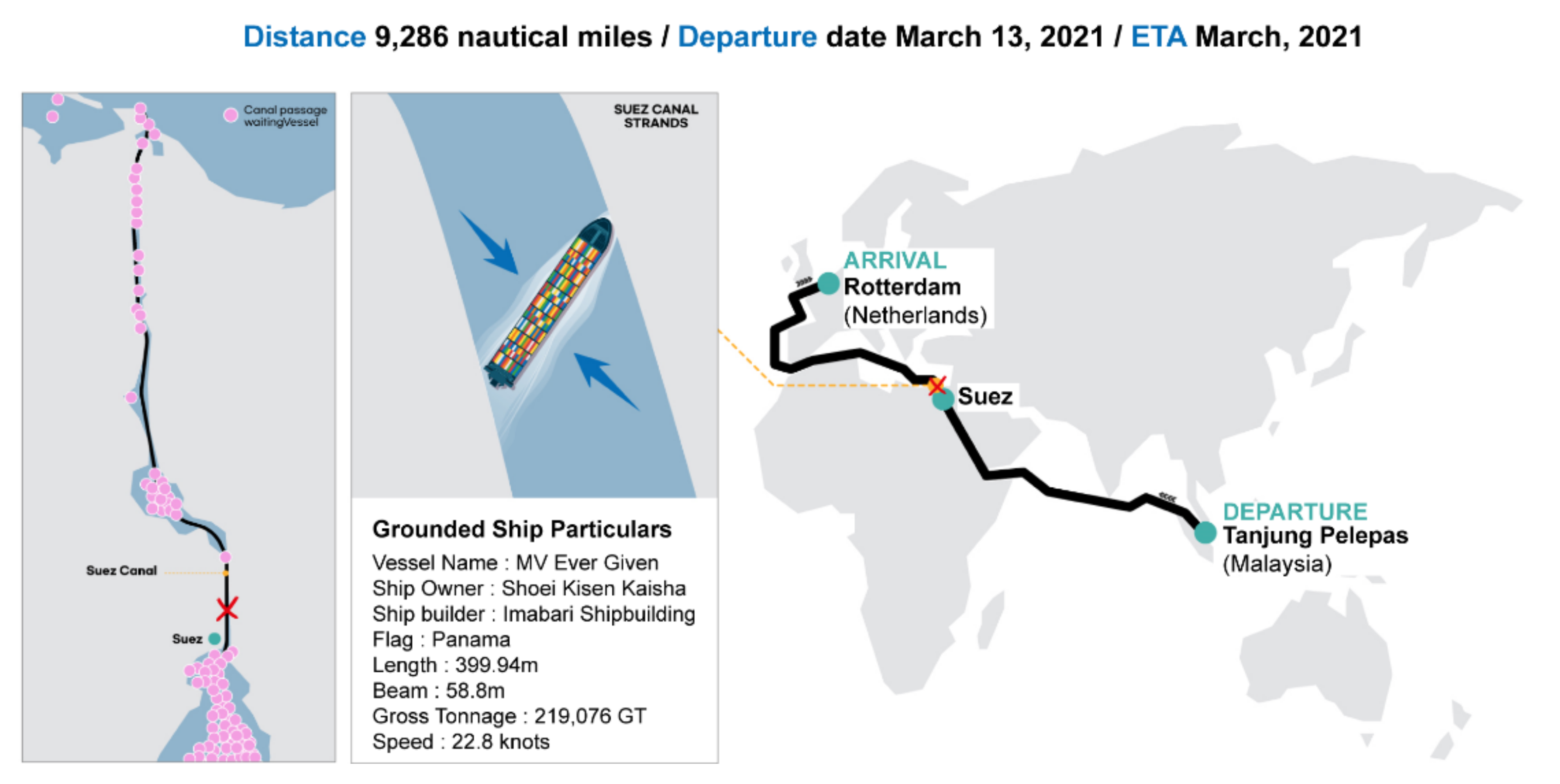This detailed diagram displays the journey and unfortunate incident of the container ship M.V. Ever Given, which became famously lodged in the Suez Canal. The diagram is divided into several sections to convey various pertinent details:

At the top, text reads: "Distance: 9,286 nautical miles / Departure: March 13, 2021 / ETA: March 2021." 

On the left side, an infographic highlights the Suez Canal showing a sequence of vessels in a vertical layout. The diagram features a red "X" indicating the precise location where Ever Given got stuck, halting traffic and causing a backlog of vessels marked in pink.

Adjacent to this, another detailed diagram depicts the vessel sideways within the canal with annotations: "Suez Canal Strands." Beneath, ship particulars include:
- **Vessel Name**: M.V. Ever Given
- **Ship Owner**: Shoi Kisen Kaisha 
- **Shipbuilder**: Imabari Shipbuilding 
- **Flag**: Panama
- **Length**: 399.94 meters
- **Beam**: 58.8 meters
- **Gross Tonnage**: 219,076 GT
- **Speed**: 22.8 knots

To the right, a large map traces the planned route of the Ever Given. The ship's journey originates in Tanjung Pelipas, Malaysia, navigates beneath India, crosses the Suez Canal, and then continues through the Mediterranean Sea, skirting the European coastline, ultimately arriving at Rotterdam, Netherlands. Detailed markers identify key waypoints and the incident point within the Suez Canal.

Overall, this comprehensive diagram visually and textually narrates the voyage, incident, and technical specifics of the Ever Given, shedding light on its extensive journey and the critical point where it disrupted a major global trade route.